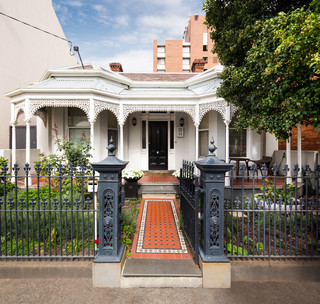The image showcases the entrance of a single-story, white house with a red sloping roof and a black door. The entrance is framed by two ornate black pillars and matching wrought iron railings that separate the sidewalk from the garden areas on either side. These gardens are lush with various green plants and there's a prominent tree to the right. A path paved with red, possibly orange tiles leads from the open gate to the door. The house stands on a portico upheld by thin, white columns. Behind the house, there's a pink skyscraper and a tan-colored building wall, noticeable on the left of the image. The sky above is a bright blue with a few clouds, adding to the architectural charm of the scene.